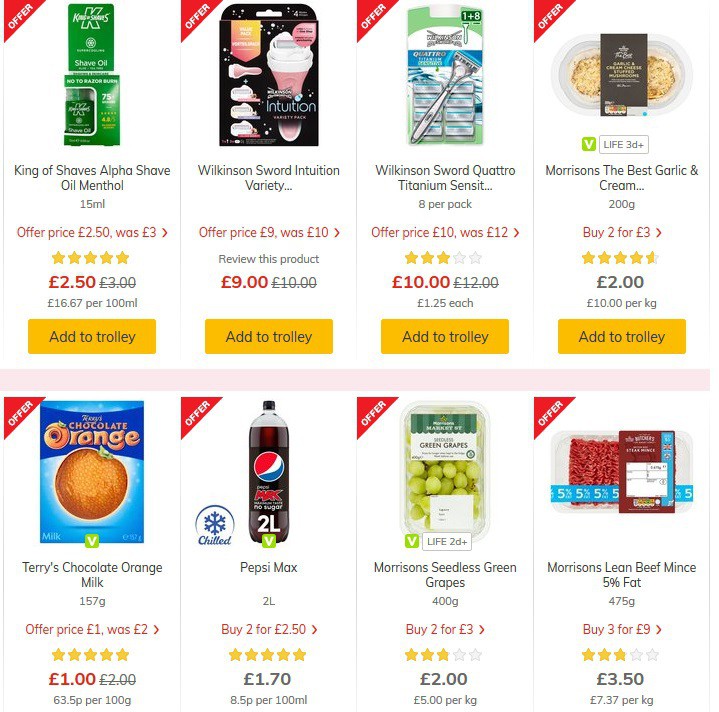The image captures a screen from an online shopping app, displaying eight different products with their respective prices. The products are arranged in two rows, with four items in each row. Starting from the top left corner, the first product features green packaging with a price of £2.50 displayed in red text underneath. Next to it, the second product comes in pink and black packaging. The third product, to the right, is presented in green, white, and blue packaging, with a price of £10 also indicated in red text below it.

In the bottom row, the first product on the left is labeled "Chocolate Orange," and is packaged in blue and orange. Next to this, moving to the right, is a clear bottle of Pepsi Max. The bottle's label is printed in white text, and it holds 2 liters of the brown-colored beverage.